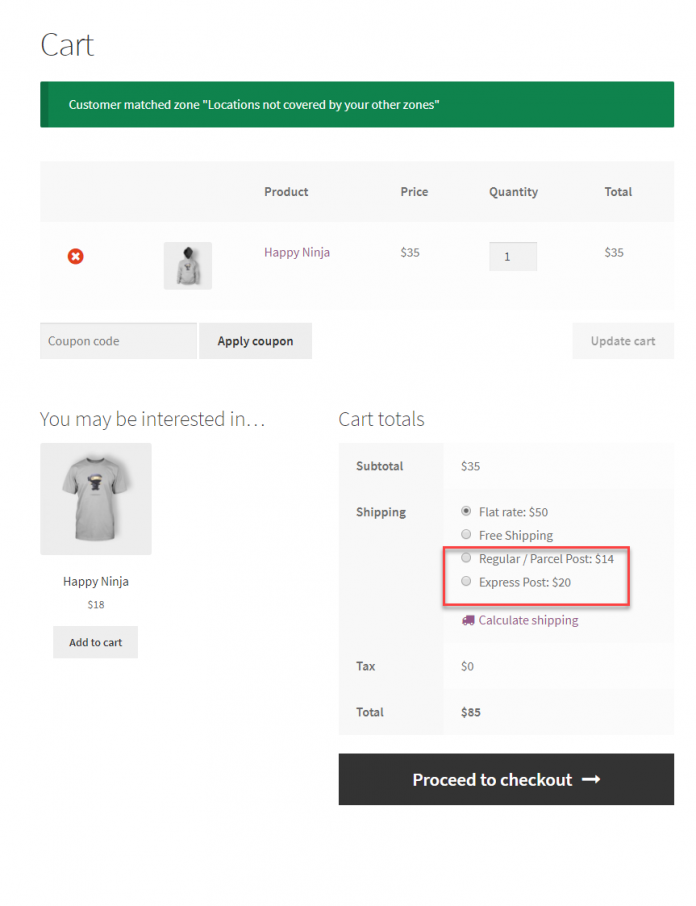**Screenshot of a Website Pop-Up Menu Detailing a Shopping Cart**

The screenshot captures a pop-up menu on a website focused on a user's shopping cart. The background is predominantly white, with "Cart" written in a large gray font in the upper left corner. Below this header, a horizontal green rectangle with white font displays the message: "customer matched zone: 'locations not covered by your other zones'."

Following this is a white navigation bar, and beneath it, a darker off-white rectangle lists the headers: "Product," "Price," "Quantity," and "Total" in dark gray font.

The product selection begins with a small red circle featuring a white "X" on the left side, accompanied by a thumbnail image of a gray hoodie sweatshirt. The product is labeled "Happy Ninja" in gray font, priced at $35. A gray square next to the price shows a quantity of "1," leading to a total cost of $35.

Below the product details, there's a section for applying discounts. A gray rectangle labeled "Coupon Code" is beside another gray rectangle with black font stating "Apply Coupon." Further to the right, another gray rectangle with gray text offers the option to "Update Cart."

At the bottom left, a recommendation section suggests additional products. It reads "You may be interested in:" in gray font, alongside a thumbnail image of a gray t-shirt.

This comprehensive pop-up effectively summarizes the shopping cart's contents and offers clear options for updating the cart and applying coupons.